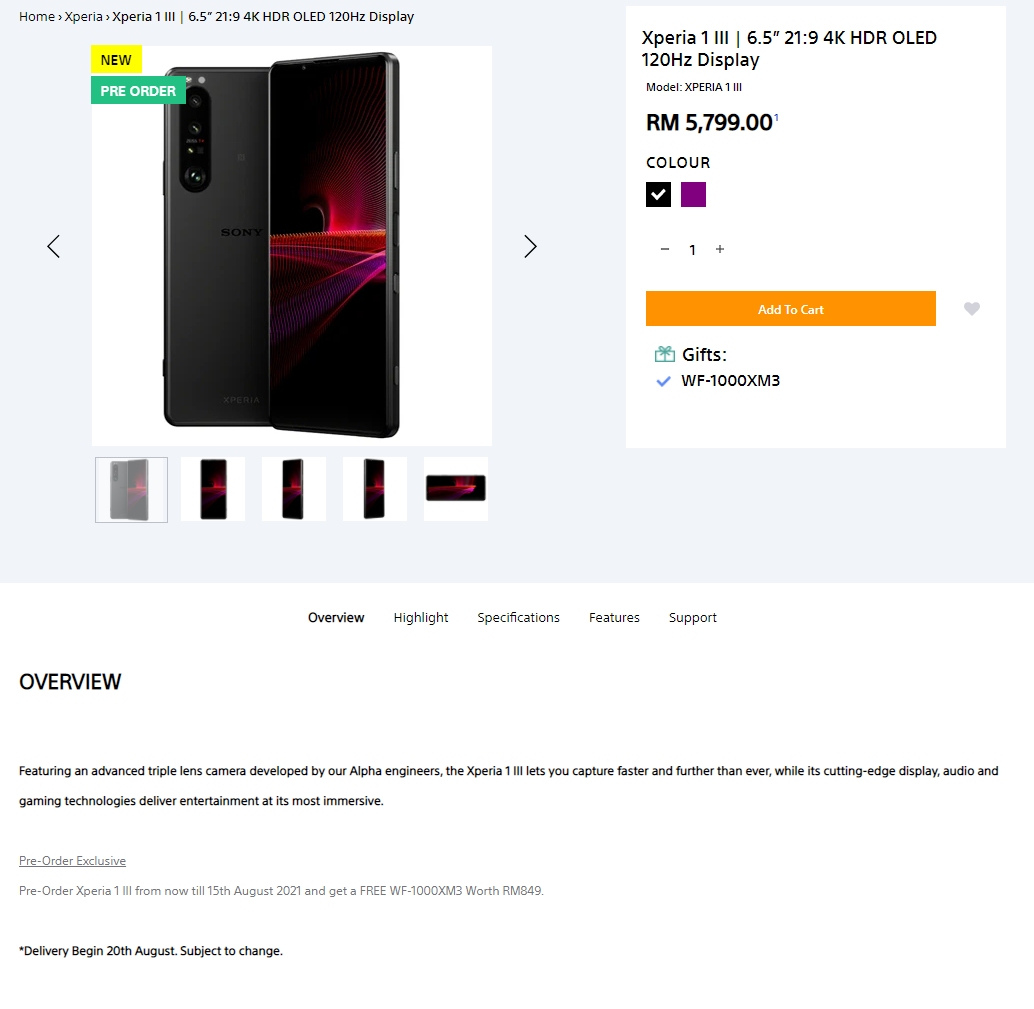This image displays a shopping page for a high-end cell phone, set against a gray background. The layout is in landscape orientation with central white boxes. At the top, in clean black font, the text reads: "Home > Experta > Experta I --- 6.5 inches, 21:9, 4K HDR OLED, 120Hz display."

The main section features an illustrative photo of a Sony phone, depicted from two different perspectives. The phone, shown in portrait orientation, is long, rectangular, and black, with the camera positioned along the left edge. The first angle reveals the phone's back, while the second angle shows the front screen, tilted slightly to create a V shape together with the back view. The screen displays a black background adorned with purple, pink, red, and orange lights.

Directly beneath this main image, there is a strip of additional photos showcasing the phone from various angles, enabling users to sift through them. On the right side of this section, another white box provides the phone's details: the model name and a price tag of RM 5,799. The section also includes options to select the phone's color—either black or purple—and the quantity to be purchased. Below this, a long rectangular orange button with yellow-white text offers the choice to "Add to Cart," alongside an option to add the item to favorites.

Further down are navigation tabs for different sections: Overview, Highlights, Specifications, Features, and Support. The "Overview" tab is currently selected, summarizing the primary details of the phone.